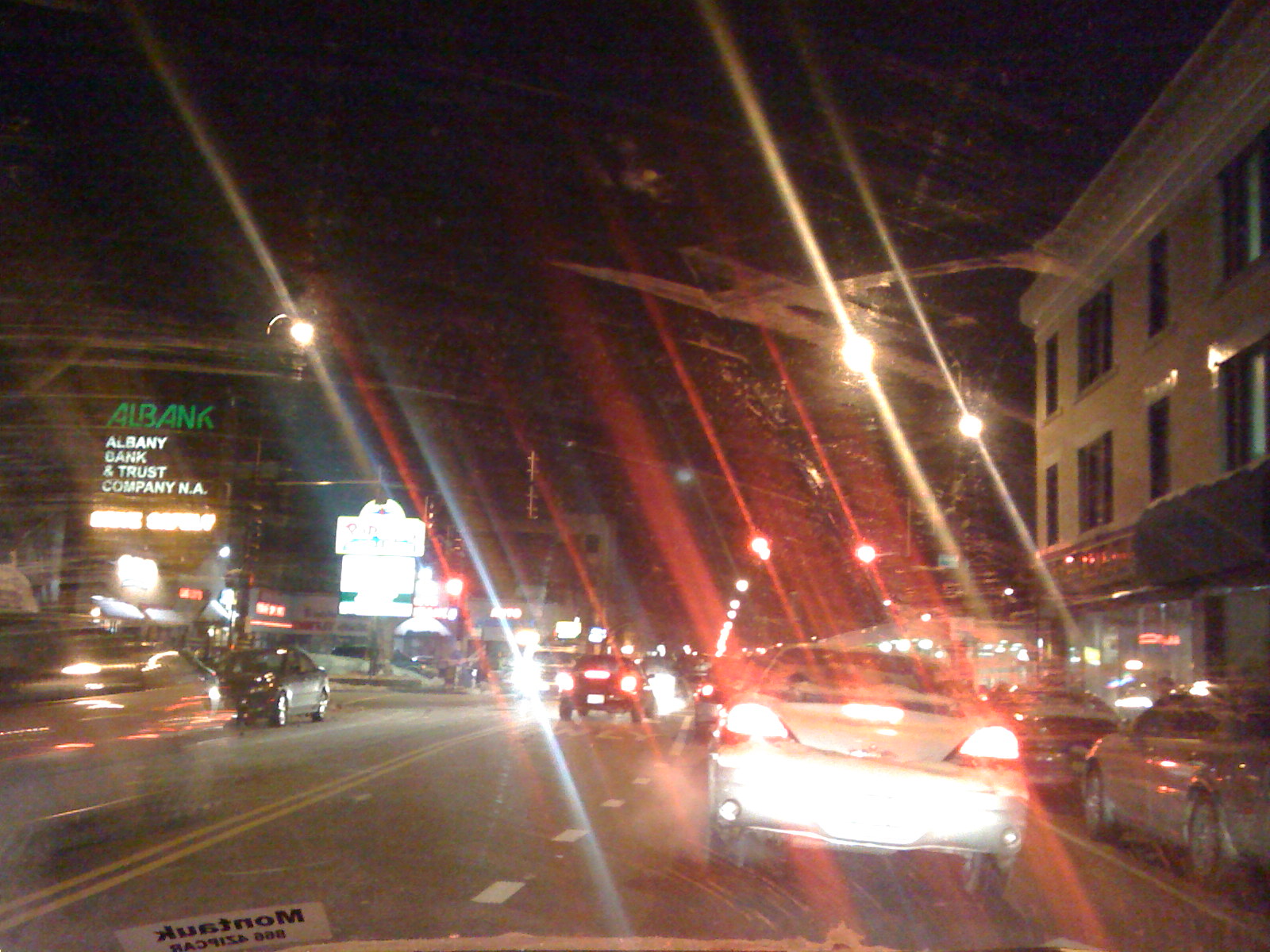The photograph captures a bustling city street at night, viewed from inside a car. The scene is illuminated by an array of streetlights and car lights, creating vibrant streaks of yellow, white, and red across the image. It is a two-way street, with cars traveling in both directions. The vehicles heading away from the camera have their brake lights on, casting a red glow, while the cars approaching are blurred, suggesting motion. Parked cars line the sides of the street, adding to the urban landscape.

On the right side of the street stands a three-story building with a storefront on the ground level and what appear to be offices above. On the left side, there's a prominent sign that reads "Albany Bank and Trust Company NA." Further in the background, more neon lights blur together, enhancing the dynamic city atmosphere. The photo, taken through a car windshield, features a partial sticker in the bottom left corner with the word "Montauk" visible, adding a layer of authenticity and personal perspective to the scene.